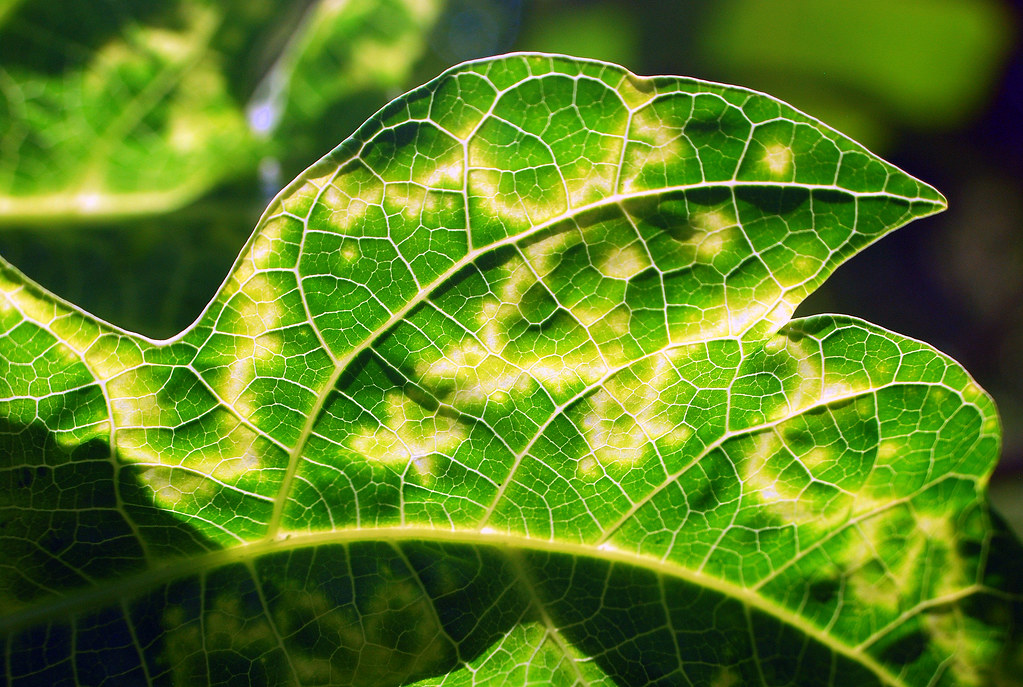This image is a horizontally aligned close-up photograph of a beautifully intricate leaf, showcasing its detailed structure. Dominating the center, the leaf's stem curves gently from the left side of the frame, leading down to the lower right. The leaf itself is an array of lively colors, predominantly bright green with sections of light green and striking patches of bright yellow arranged in a zigzag pattern.

The leaf has a scalloped edge and is partially shadowed, indicating sunlight filtering through, which creates a play of light across its surface. Its veins, pronounced and whitish, spread throughout, adding to the elaborate texture. The top edge of the leaf curves up towards the upper right, forming a pointed tip, while the bottom edge angles downward, culminating at the bottom right corner of the frame.

The background is a blurred expanse of similar foliage, suggesting a lush environment, but it is indistinct, drawing the focus entirely to the leaf in the foreground. On the right side of the image, the background is darker, contrasting with the lighter hints seen on the left. Additionally, a blurred representation of another similar leaf is discernible in the upper left corner, mirroring the highlighted and shadowed interplay seen on the focal leaf. This detailed close-up vividly captures the leaf's textured beauty against a softly blurred backdrop.